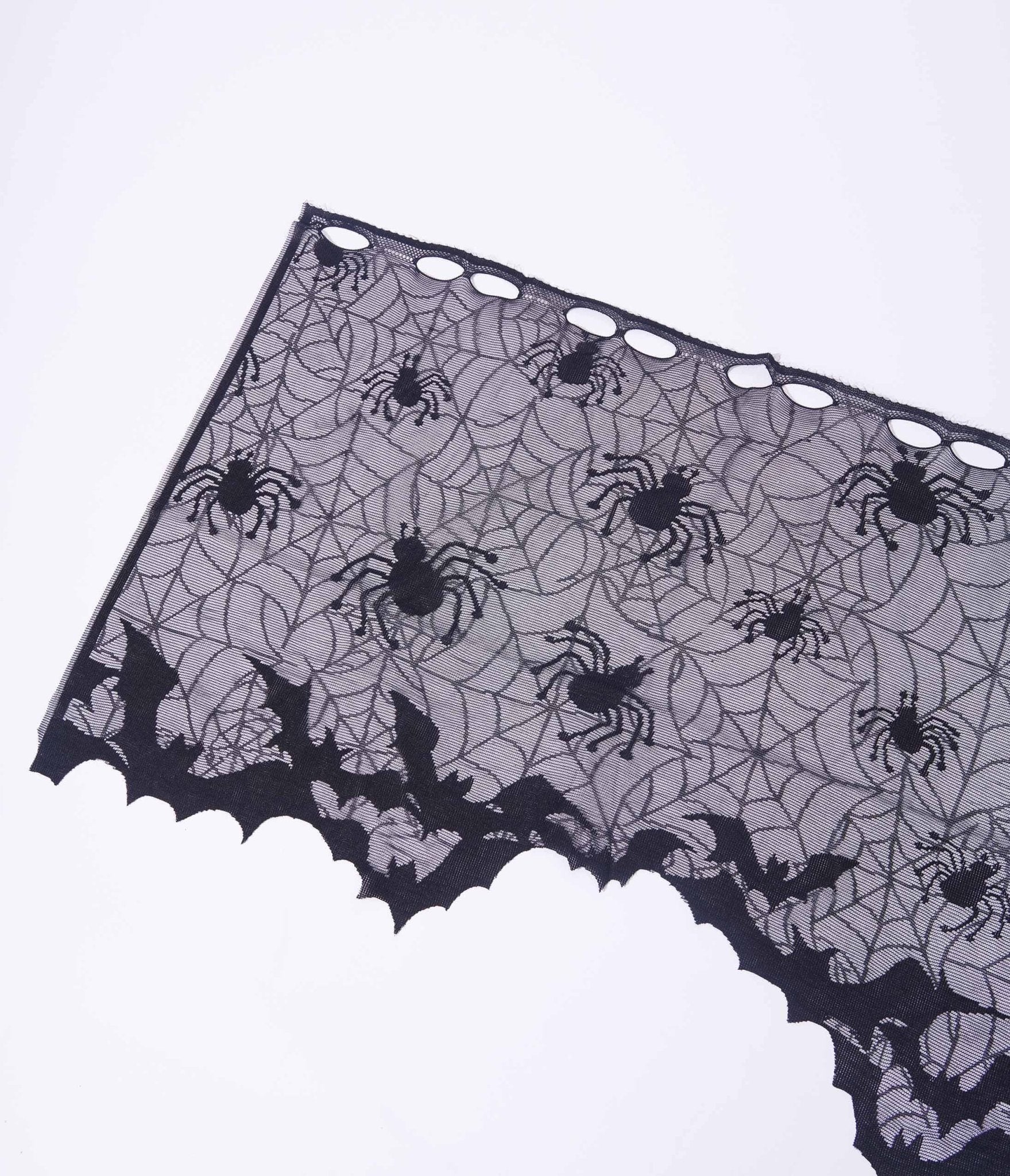This image is a close-up, black-and-white photograph of a Halloween-themed valance or curtain. The valance is designed to adorn the top section of a window, characterized by its decorative and festive aesthetic. The fabric is adorned with an intricate pattern of spider webs and spiders of varying sizes, some descending from the webs. At the top, the valance features evenly spaced holes intended for threading a pole or curtain rod. The bottom edge of the fabric is creatively cut and shaped to resemble bat wings, accompanied by additional bats flying just above this area. The overall scene, which is printed on a gray fabric, combines elements like diamond patterns integrated with spiders and webs, creating a spooky yet playful Halloween motif. The background of the image is a light gray, highlighting the contrasting dark, cartoonish illustrations.